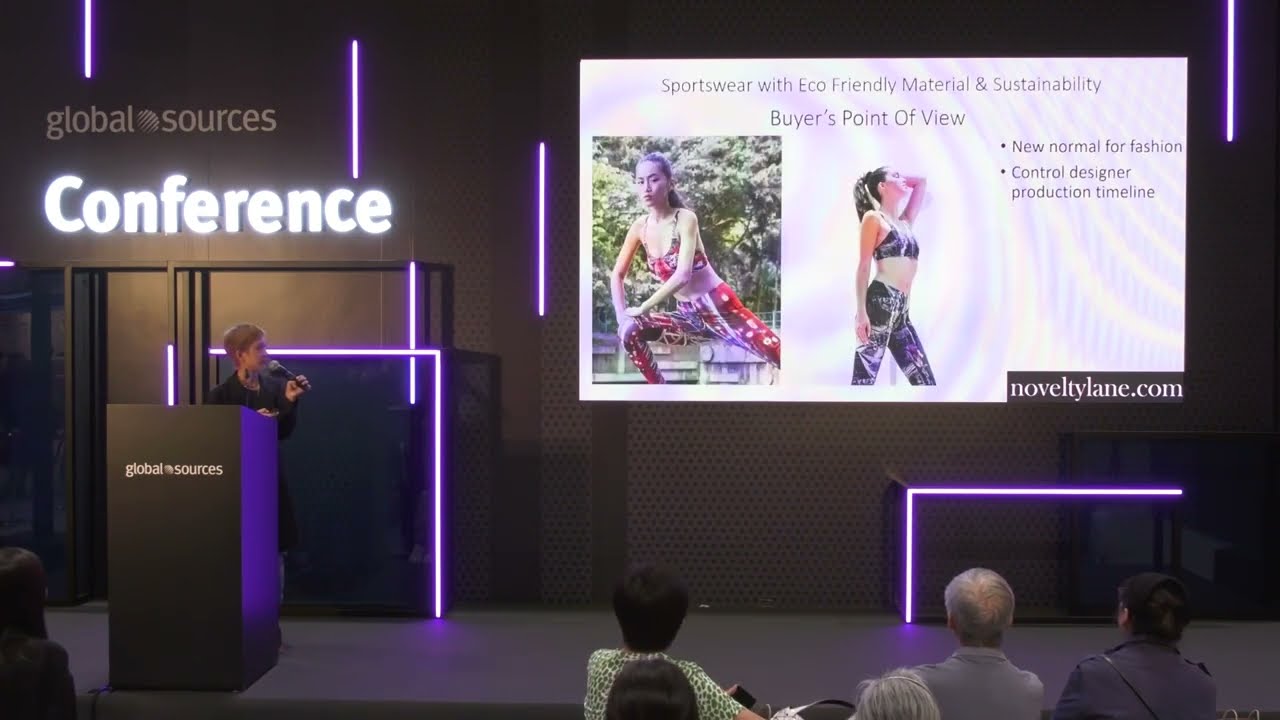The image depicts a Global Sources Conference, captured in a landscape format, approximately one and a half times wider than it is tall. At the bottom, the heads of several middle-to-elderly audience members are visible, attentively watching the stage. The stage has a brownish-gray backdrop and features a black podium on the left, prominently displaying the words "Global Sources" in white lettering. A middle-aged woman, holding a microphone in her left hand, stands behind the podium and is speaking, possibly discussing what's shown on a screen to her right. 

The screen, positioned in the upper right-hand corner of the image, displays content from a projector. At the top, the slide reads "Sportswear with Eco-Friendly Material and Sustainability, Buyer's Point of View." Two bullet points follow: "New Normal for Fashion" and "Controlled Designer Production Timeline." The screen features images of two women. The first, on the left, is a young woman in red and multicolored workout gear, captured in a forward lunge with her hands on her knees. The second, in the center, is a fit woman in a black sports outfit, comprising bottoms and a bra-like top, looking upwards, her hair tied back in a ponytail. The slide also includes the text "noveltylane.com."

Adding to the scene, purple neon lights frame the stage, providing a modern and dynamic ambiance.